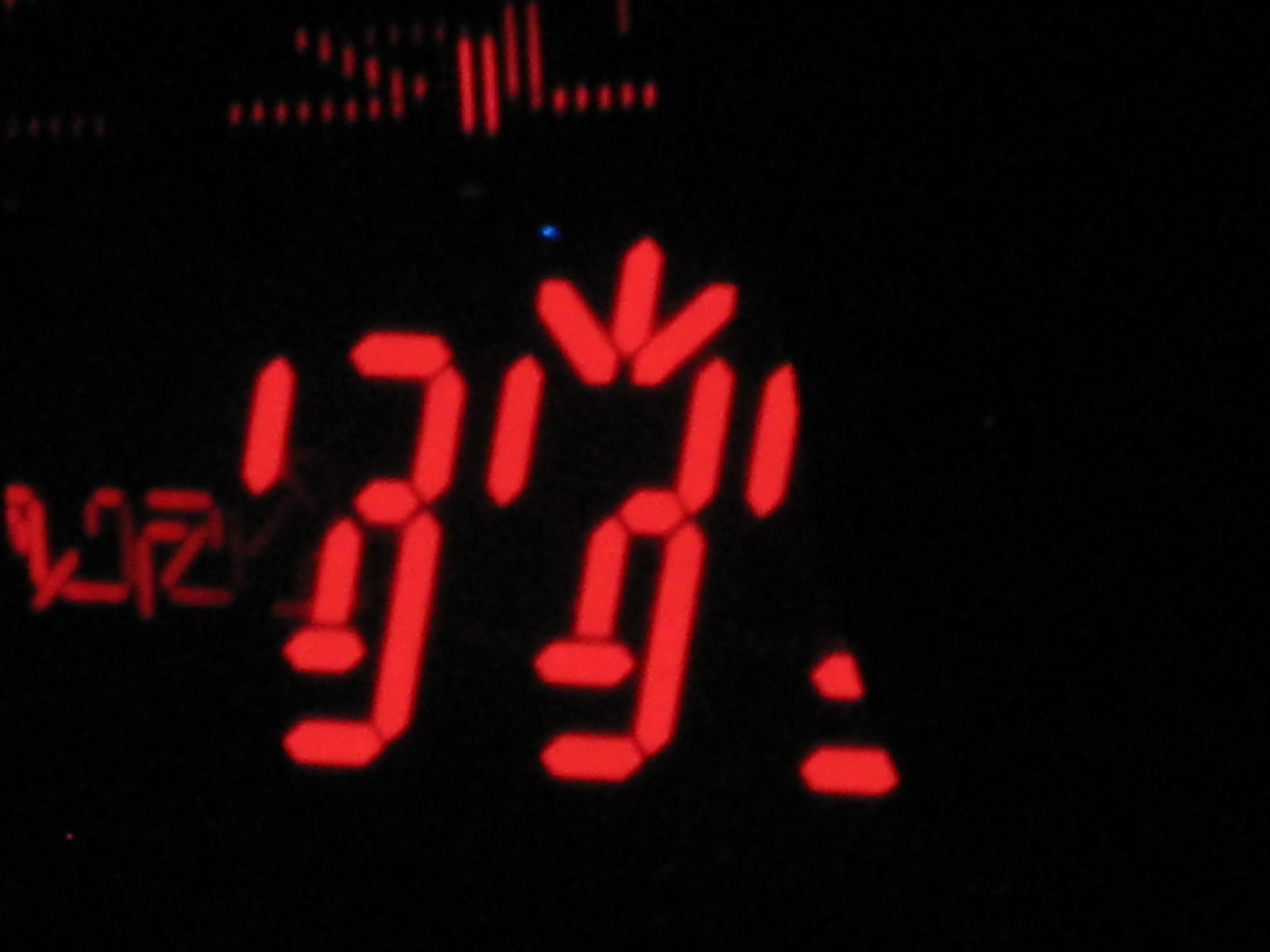The image appears to be a very dark depiction with an entirely black background that prominently features red, LED-like, digital clock numbers. These red segments resemble numbers but don't form coherent figures, giving the impression of either a malfunctioning device or a blurred photograph taken while in motion. The numbers are reminiscent of the design found on the cover of The Police's album "Ghosts in the Machine," where red digital number-like shapes symbolically represented the band members against a black background. Additionally, there are sporadic red dots and lights in the upper left area and along the left side, further enhancing the chaotic, glitch-like aesthetic. Overall, the image exudes a sense of disarray, suggesting either a faulty electronic display or the effect of camera movement capturing a fragmented, digital time display.